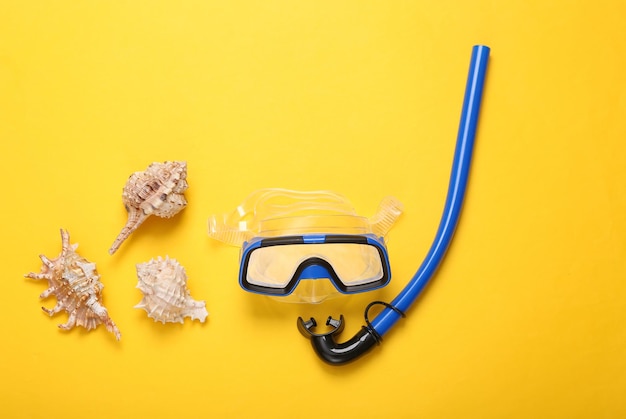The photograph features a vibrant, high-saturation yellow background, reminiscent of toy-like primary colors. Central to the image is a set of scuba gear: a diving mask framed with blue and black edging and a snorkel positioned beneath it. The snorkel has a blue tube with a black base. To the left of the scuba gear, three seashells are arranged in a triangular formation. The seashells vary in appearance, with one appearing spiky, another with a thin top and a bulbous end, and the last resembling a pufferfish. Their colors range from whitish to grey with spotted patterns, incorporating hints of light brown, tan, red, and pink.